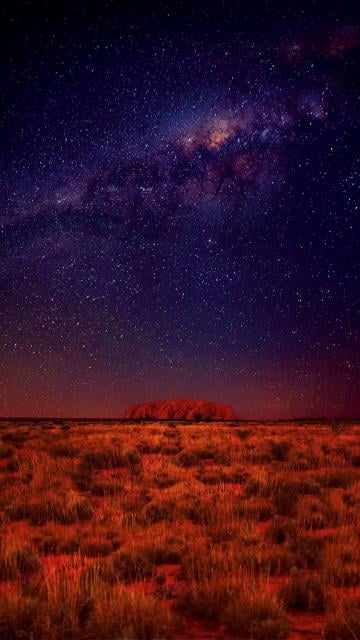This vertical, rectangular-shaped photo, taken at night, features a dramatic, otherworldly landscape that blends science fiction elements with natural beauty. The sky is predominantly a deep bluish-black with an abundance of stars densely clustered together, evoking a sense of a vast cosmos. Interestingly, there are shades of red and purple among the stars, enhancing the otherworldly atmosphere.

The ground in the photo is strikingly red, reminiscent of the Martian surface, stretching out like an expansive, empty field. This reddish terrain, possibly dotted with high grass or distinct red plants with dark sage or smoky green stalks, adds to the alien-like ambiance. The horizon features subtle earth-tones, with a red hill and hints of brown, transitioning into the star-filled sky.

Overall, the image creates a beautiful, almost surreal scene where the dark, bluish night sky contrasts with the reddish, earthly foreground, culminating in an imaginative and visually captivating landscape.